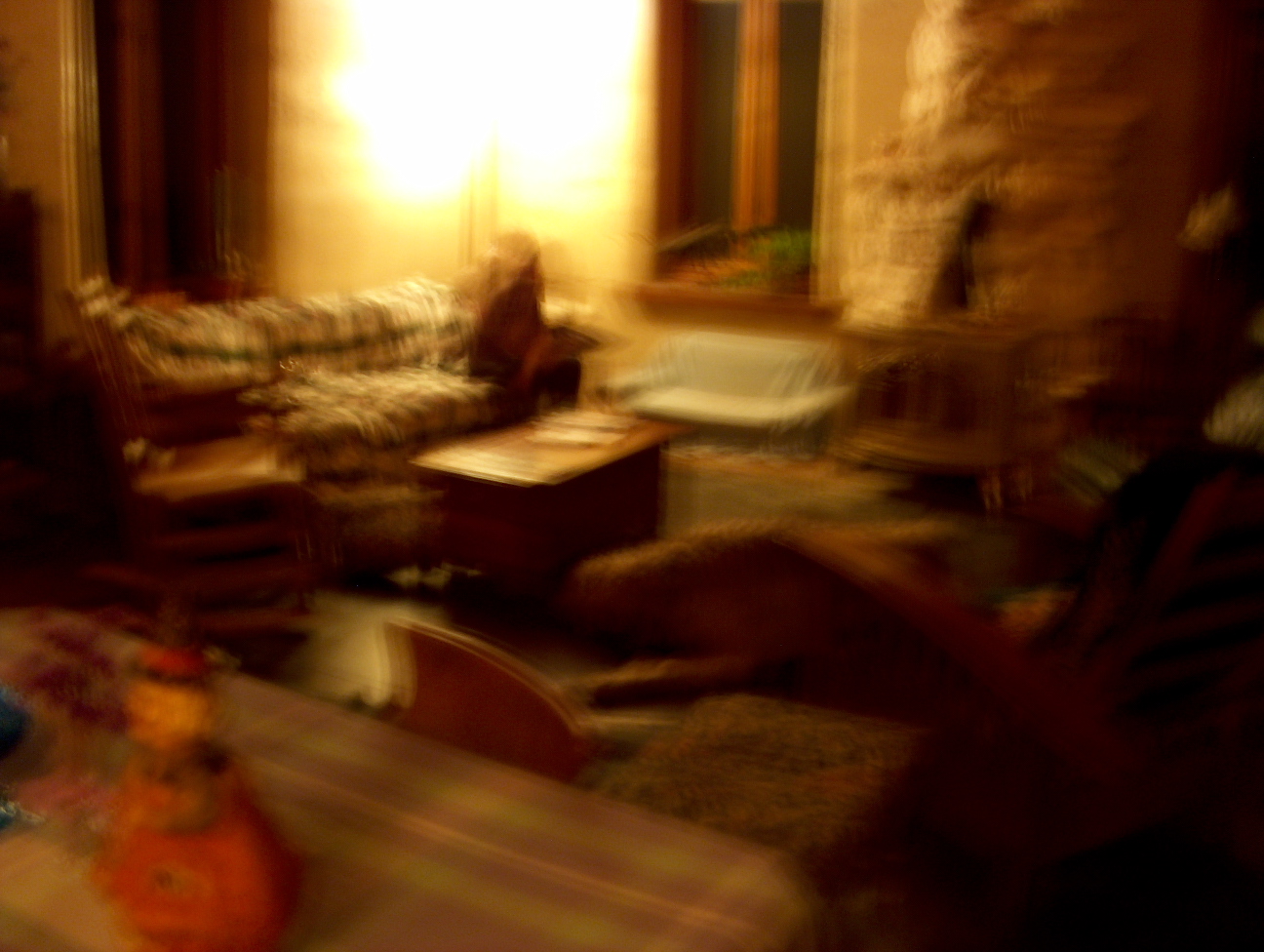The image depicts a very blurry and out-of-focus photograph of a cozy, possibly nighttime, family or sitting room. At the center of the scene, a glowing light fixture casts a strong illumination throughout the space. On the left side of the image, a white and green-striped three-seater sofa features an older gentleman with a bit of white hair sitting on it, while a rocking chair is positioned nearby. To the right of the sofa, a brown coffee table or trunk is placed on the wooden floor, along with a possible gray, half-shaped object. Near this table is a creamy-colored dog that could be a golden retriever or Labrador, lying with its legs stretched out. At the forefront, there's a smaller striped table with green, red, and yellow detailing, adorned with a doll in a red skirt. The room also contains a few stools, additional tables with various objects, and a window with a wooden frame from which the glowing light originates, completing the warm and homely atmosphere of the space.